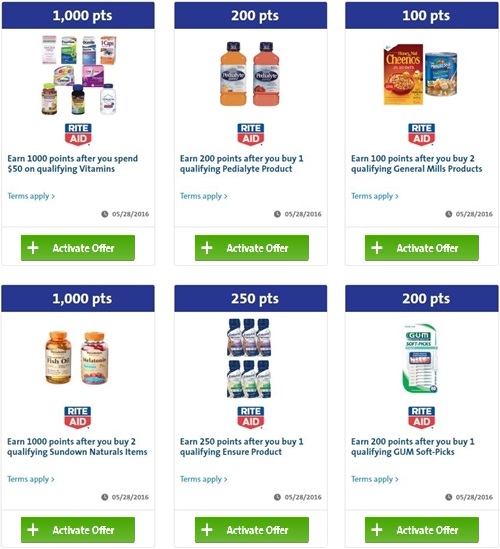This is an image of a rewards offer page, presumably from a desktop or mobile device. The page showcases six promotional offers, each designed to allow users to earn points by purchasing specific products from Rite Aid. 

Starting with the top-left offer, a blue banner reading "1,000 points" appears above images of various vitamin products. The detailed description below the banner states, "Earn 1,000 points after you spend $50 on qualifying vitamins." A green button labeled "Activate Offer" is shown at the bottom.

To the right, another offer features a blue banner with "200 points" displayed above two bottles of Pedialyte. The accompanying text reads, "Earn 200 points when you buy one qualifying Pedialyte product," with a green "Activate" button below.

The third offer on the top row has a blue banner indicating "100 points." It shows a picture of Honey Nut Cheerios and a container of soup. The description explains, "Earn 100 points after you buy two qualifying General Mills products," and includes a green "Activate" button at the bottom.

On the bottom-left, there's an offer displaying images of two bottles of vitamins. The caption reads, "Earn 1,000 points when you buy two qualifying Sundown Naturals items," and it also features a green "Activate" button at the bottom.

Next to it, another offer displays what appears to be bottles of Ensure beneath a "250 points" banner. The offer details state, "Earn 250 points after you buy one qualifying Ensure product," with a green "Activate" button at the bottom.

Lastly, to the right, is an offer with a blue banner that says "200 points" above an image of dental flossers labeled as Gum Soft-Picks. The description reads, "Earn 200 points when you buy one qualifying Gum Soft-Picks," and a green "Activate" button is located at the bottom.

Each offer is neatly presented with clear instructions on how to earn the points, emphasizing the types of products and the quantity required for each reward.